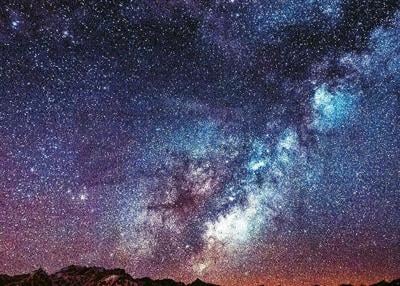This high-definition photograph captures a mesmerizing night sky filled with a multitude of stars. The sky transitions from a deep black at the top to varying shades of blue, purple, and pink towards the horizon. Central to the image is a vibrant section, possibly part of the Milky Way, emitting a blend of white light and magenta hues intertwined with swirling black clouds. The scene is grounded by the silhouettes of rugged mountain peaks at the bottom, accentuating the celestial display above. The entire composition gives the sky an almost textured appearance, as if colored sand has been spread across the heavens.